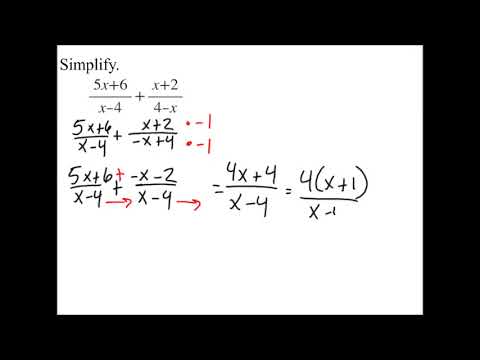The image features a striking black border that frames the entire composition. Within this black frame, there is a secondary, thick gray border on the left and right sides, creating a stark contrast with the central area. Dominating the center is a bright white square resembling a piece of paper, set against a slightly darker, grayish-white background. At the upper left corner of the paper, the word "simplify" is written in a computer-style font. Below this directive are intricate, handwritten mathematical equations, forming a complex problem involving fractions with variables and subtraction. The equations have been meticulously worked out in a sequence, mostly in black ink, while approximately 10% of the notations are in red ink, indicating corrections or additional notes. Red parentheses, arrows, and other symbols emphasize specific parts of the equation. The ultimate simplification results in the expression -x². The image's overall layout, with its black, gray, and white elements, evokes a sense of structured academic rigor, akin to a detailed problem-solving exercise seen on a chalkboard or paper in a math classroom.